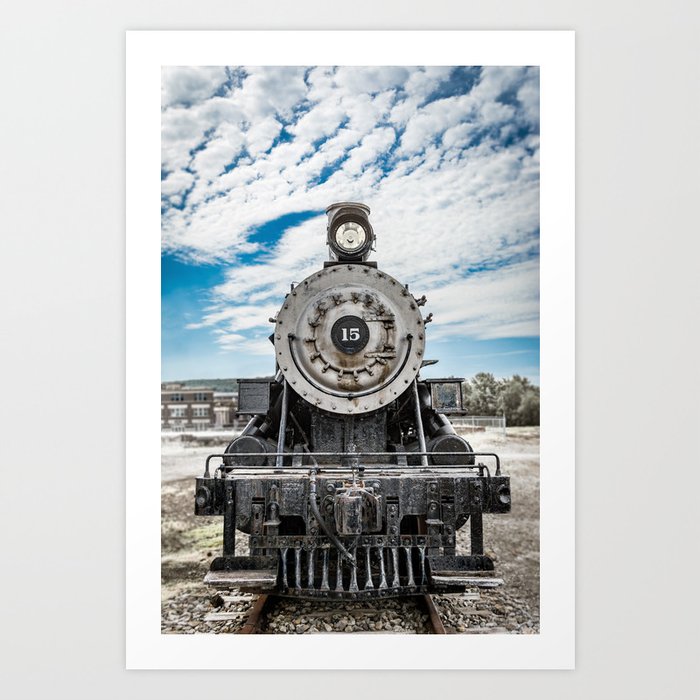The image captures a full-color, head-on photograph of the front of an old train engine, prominently displaying the number 15. The train is black with silver and chrome details, though a layer of white dust or frost suggests age and weathering. Sitting on a bed of small stones on the tracks, it stands out as the main focal point against a bright blue sky adorned with puffy, white clouds. To the left, slightly blurred, are old train cars in a yard, while the right side features a backdrop of trees. The ground around the tracks includes frost-tinged grass, adding to the sense of a crisp, possibly cold, day. Various pipes and metalwork are visible, showcasing the intricate details of this classic train.